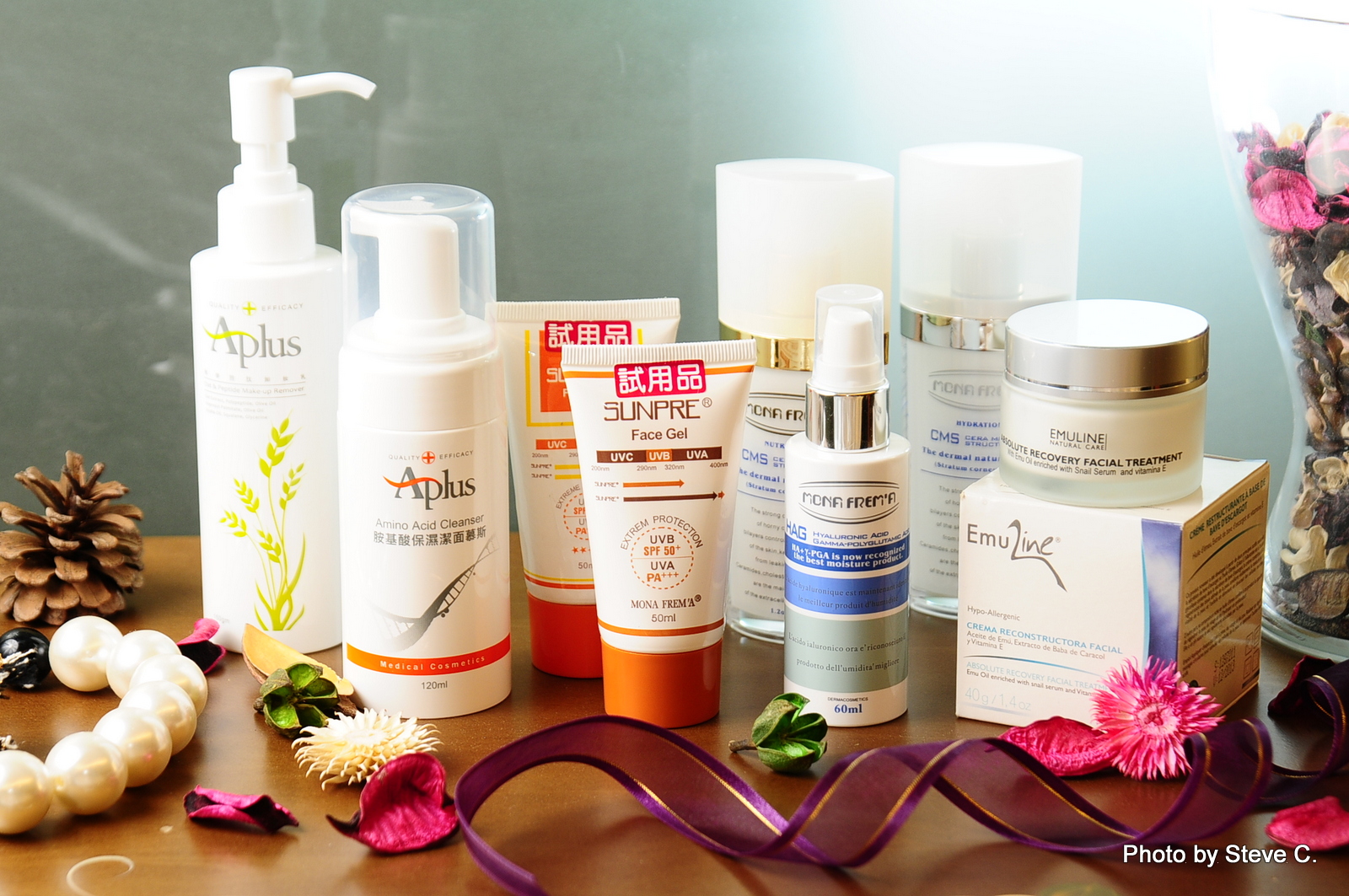This is a color photograph featuring a meticulously arranged set of cosmetics displayed on a reflective wooden surface. The backdrop is a muted greyish-green, with a lighter shade illuminated by light seeping in from the top right corner. A small whitish scratch is visible on the wall to the left. 

In the foreground, a coiled, purple translucent ribbon with a gold edge cascades gracefully. The bottom right-hand corner bears the white inscription, "Photo by Steve C." Towards the left corner of the table, a pinecone sits next to a string of thick pearls, likely part of a pearl necklace or bracelet. Scattered potpourri, in shades of pink, white, and green, along with various leaves and petals, adds a touch of natural charm.

The right edge of the image reveals the corner of a jar filled with similar-colored potpourri. A variety of cosmetic bottles and jars dominate the scene. On the left, a white bottle with a pump features "A+" in black and a sheaf of wheat design. Beside it, a smaller bottle also labeled "A+" with an orange rim at the bottom, showcases a similar wheat motif.

Further right, two identical sun cream tubes with "Sun Free" and possible Chinese characters in white and orange stand together, presumed to be SPF 50. Adjacent to these are three bottles with blue and white labels and large white caps, the back two being taller and identical, while the front one, slightly smaller, features a pump and a similar but smaller cap. 

Additionally, a white jar labeled "In Use Inc." in black text lies near the back, topped by a round jar with a silver top, possibly containing the product featured in the box below.

This carefully curated collection of cosmetic products, highlighted by sunlight and enhanced with decorative elements, presents an aura of elegance and refinement.